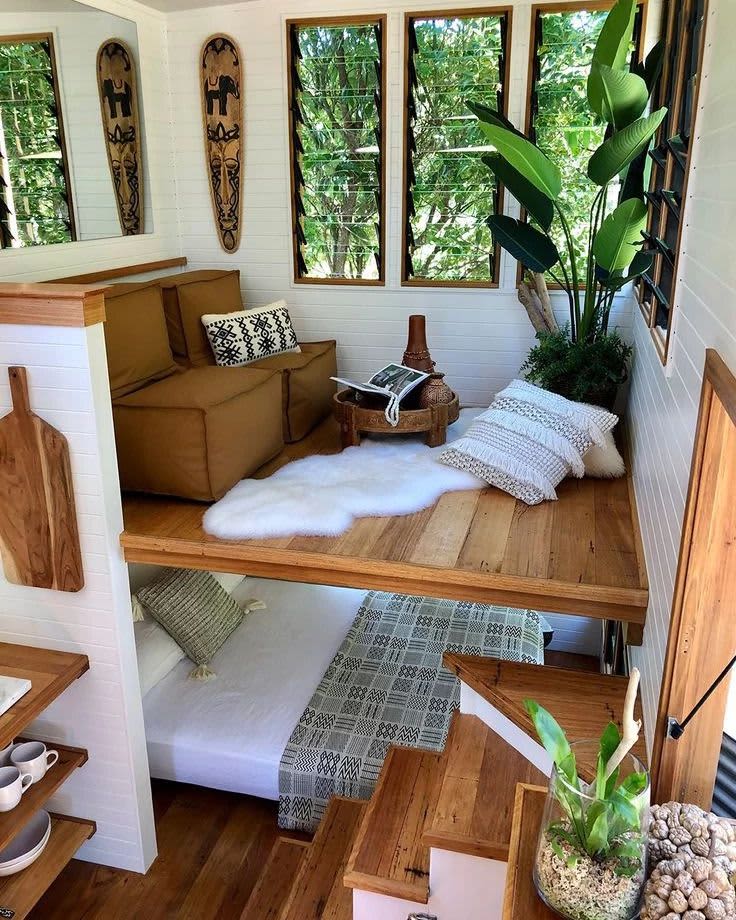This interior shot showcases a meticulously designed tiny home with an open floor plan, capturing its aesthetic and functional elements from a lofted vantage point. The home features three tall slit-like glass windows along the back wall, through which a vibrant blue sky and lush green trees are visible, enhancing the airy atmosphere. The interior boasts white-painted brick walls and rich wood flooring.

The tiny home is structured on two levels. The upper level, accessible via a set of five wooden steps with the top step uniquely triangular, is a cozy loft. This space is adorned with a soft white rug, a small wooden round table, and several throw pillows. Potted plants add a touch of greenery, while multiple slatted ventilated windows bathe the area in natural light. Two single-person chairs with brown fabric sit along one wall, inviting relaxation.

Directly beneath the loft lies a spacious bed with white sheets and a green checkered bed covering, complemented by a pair of white pillows with an additional green pillow on top. A patterned black and white blanket is neatly folded at the foot of the bed. A small, well-organized kitchen area features white tiled walls, shelves with teacups, and plates, bringing practicality into the stylish setting. The front door is located at the bottom right corner, adjacent to a set of stairs that lead to this charming, compact living space.